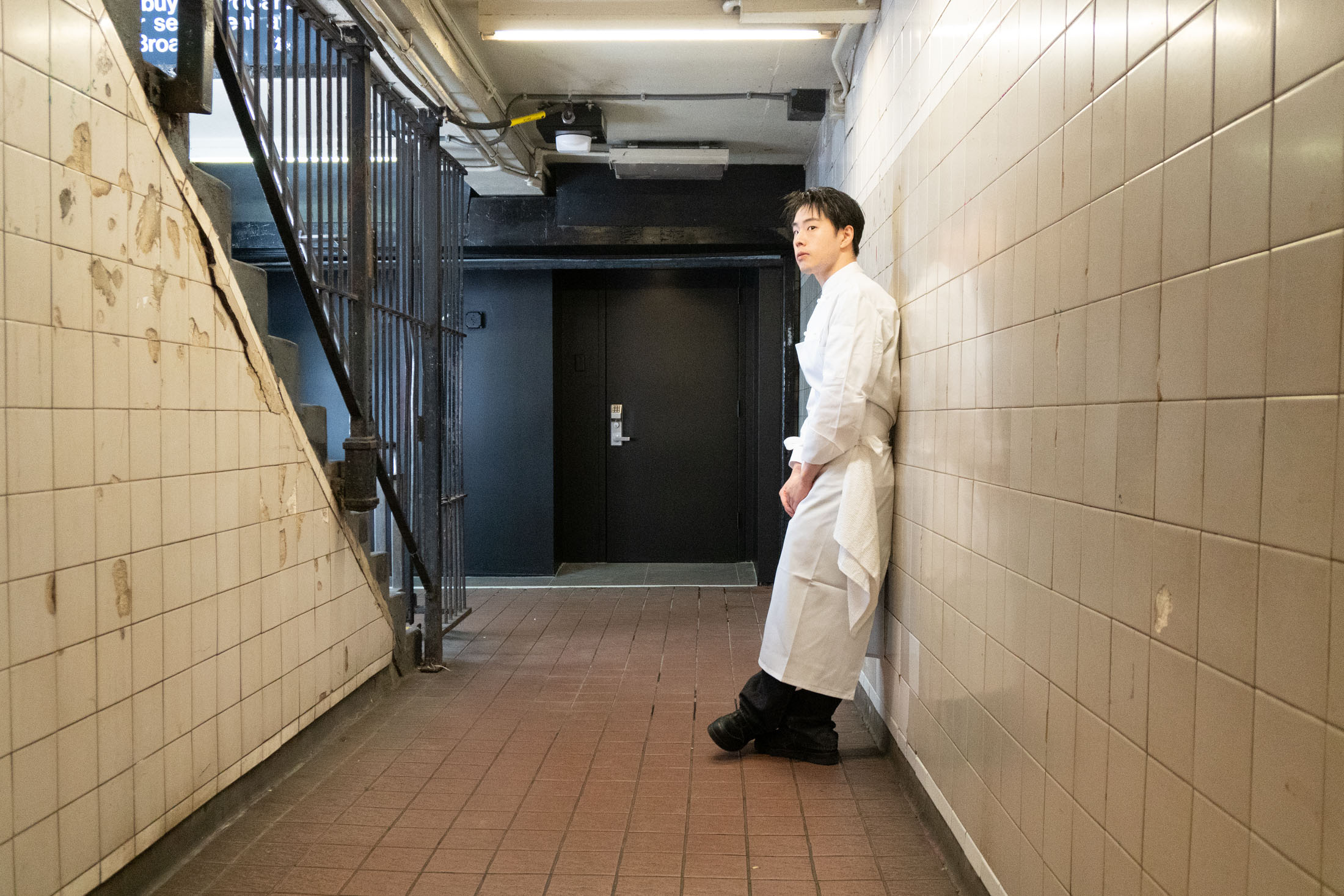In the photograph, a young Asian man, possibly in his 20s or 30s, stands in a grungy, beige-tiled hallway. He is dressed in a full white chef's uniform, which includes a long-sleeved white shirt, a long white apron that extends to his ankles, black pants, and black shoes. The man has dark hair and is leaning against a ceramic-tiled wall on the right side of the image. Directly in front of him is a staircase with a metal handrail, featuring spotted tiles at the base. The floor of the hallway is brown and appears to be made of brick. Above, industrial lighting illuminates the space. At the end of the hallway, a large black door with a lock is visible. To the left, there is part of a blue sign with writing that is partially obscured. The man gazes slightly left of the camera.